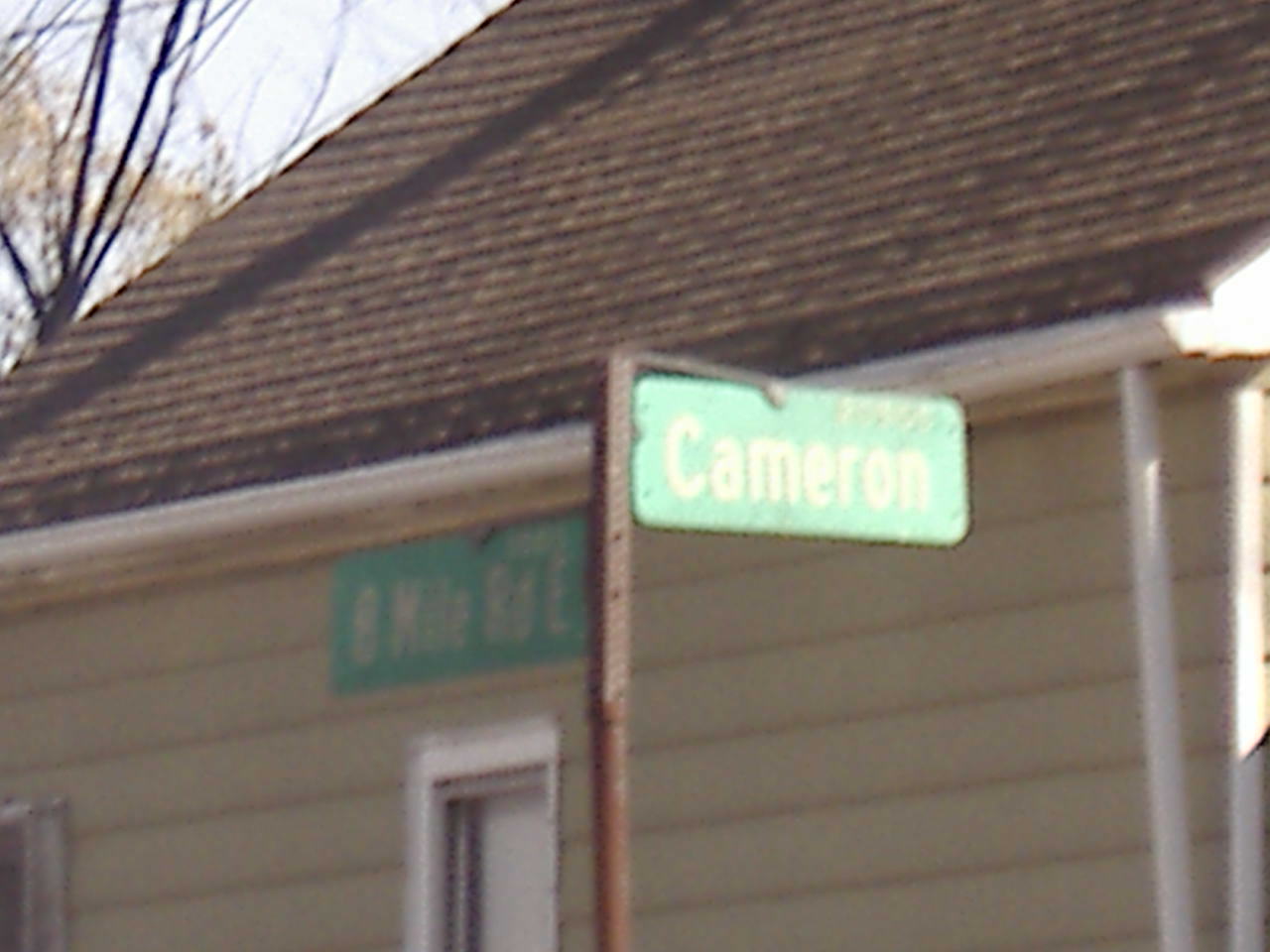The image features a basic, green street sign with white lettering that reads "Cameron." The sign is attached to a rusted pole and is positioned near a tan-colored house with a brown roof. Adjacent to the house and partially obscured, there is another street sign mounted on the wall that indicates an eastward direction, but the exact text is unreadable. The house has a white door and door frame, and above the roofline, white gutters and a water spout pipe are visible. In the background, trees can be seen extending over the house, with gray skies peeking through the foliage.